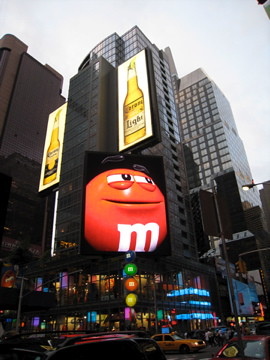This color photograph, taken in portrait orientation, captures a bustling urban landscape reminiscent of Times Square. Dominating the center of the image are three tall, dark gray skyscrapers with sleek, black glass facades. Two prominent beer advertisements are featured on the central building facing left—a bottle of Corona and Corona Light, both filled with yellow liquid. Below the Corona Light bottle, a large screen prominently displays the mischievous red M&M character, identified by its narrowed red eyelids, a white "M" on its belly, and a slit mouth. Beside the red M&M, a whimsical stoplight made of M&Ms—red in the center, yellow on the bottom, and green on the top—adds a playful touch.

At street level, vibrant and colorful lights shine from the windows of the surrounding buildings, illuminating the scene below. Bright blue lights adorn the awning of one building, and near the corner, an illustration of an orange M&M with a smile and slit eyes extends from the edge of the structure. Below these vibrant displays, cars and taxicabs navigate the busy intersection. The sky above is overcast, casting a pale, almost white backdrop that contrasts sharply with the dark towers. Reflective surfaces and neon signage give the photograph an energetic, albeit slightly blurred, atmosphere filled with motion and light.